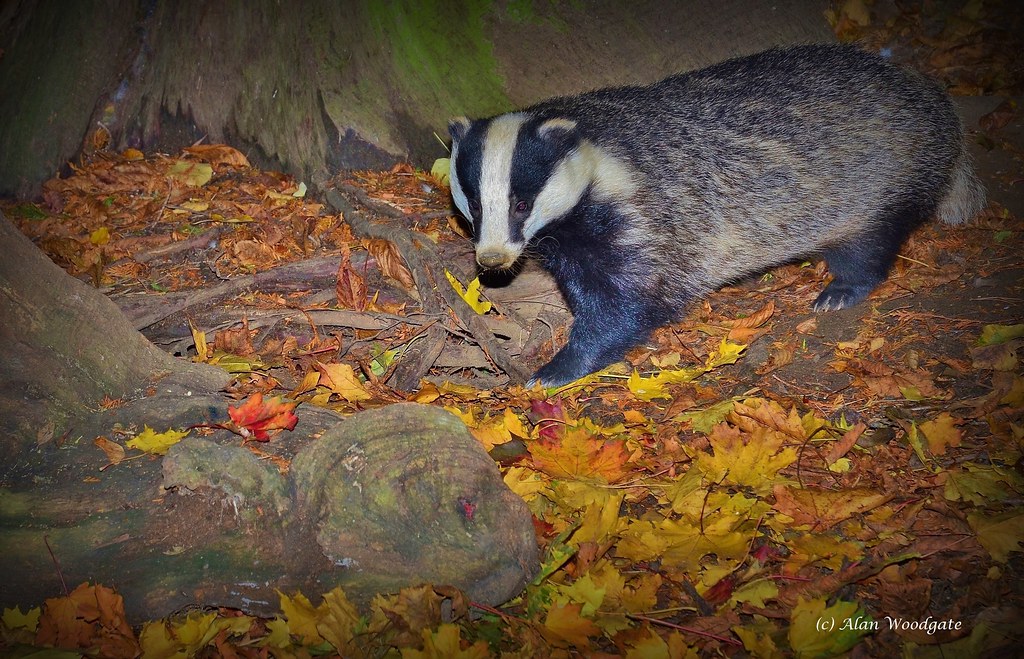In the foreground of this vibrant photograph, a long-bodied animal with a distinctive appearance roams a leaf-strewn forest floor, which is covered in colorful yellow, orange, and red leaves, indicative of the fall season. The animal, potentially a wolverine or a skunk, exhibits a striking coloration pattern: its body is predominantly grey with patches of black, and its head features black and white stripes, creating a vivid contrast. The creature's head is mostly white with a black stripe running from its ears over its eyes, giving it a unique look. Its short legs are black and end in paws with thick claws, and it has a bushy, grey tail. The animal is positioned above the littered ground, moving towards the left side of the image while curiously glancing down at a log lying in front of it. In the background, a jagged, broken tree trunk covered in moss and bark remnants frames the setting, adding to the scene's rustic charm. The photograph, credited to Alan Woodgate as noted in the bottom right corner, is brightly illuminated, suggesting it was taken with a flash, capturing every detail of this nocturnal woodland encounter.